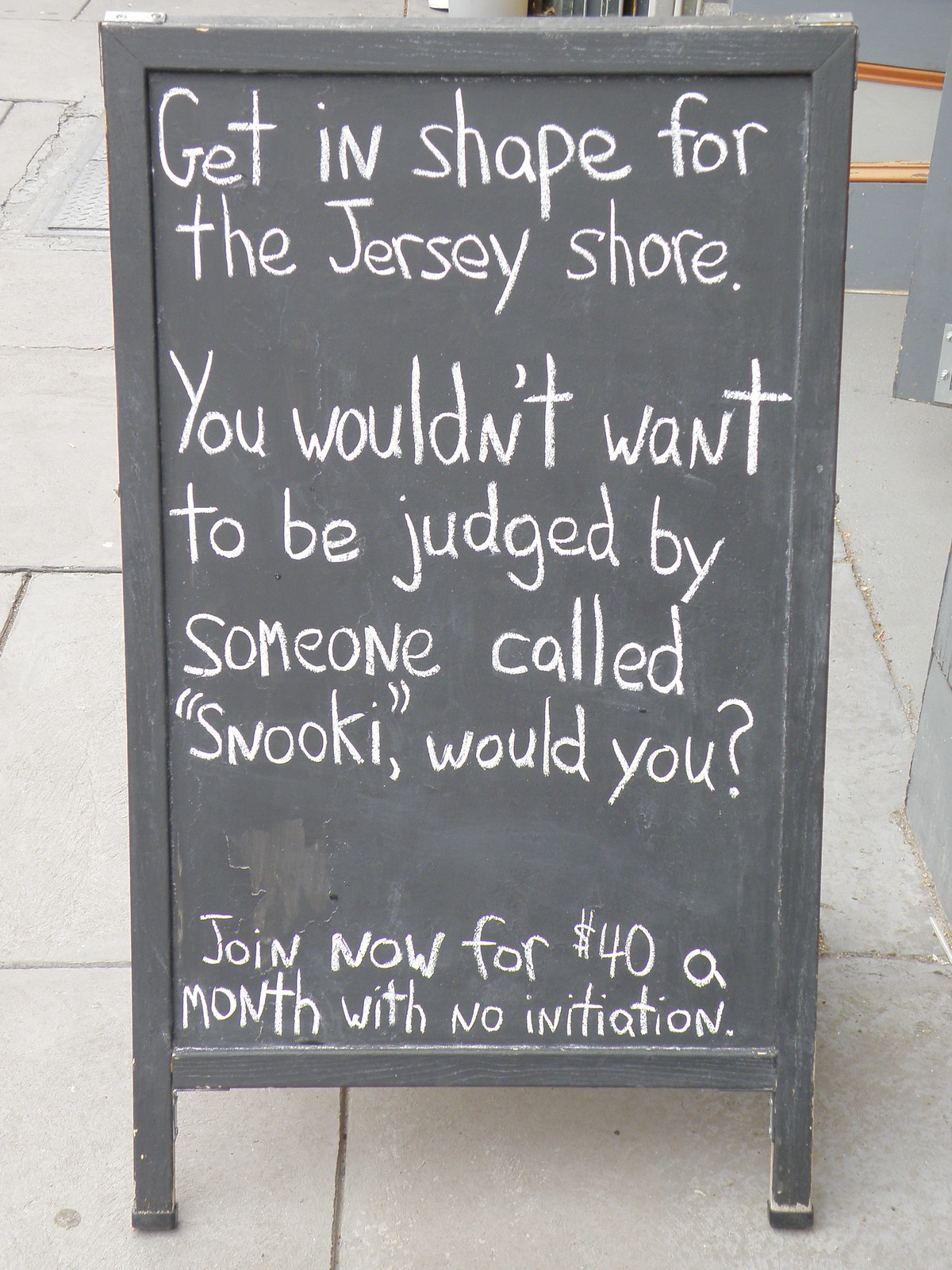The image depicts an outdoor wooden signboard positioned on a gray stone-paved sidewalk during the daytime. The rectangular, weathered, gray folding sign has a central chalkboard section with white chalk writing. The text on the board reads, "Get in shape for the Jersey Shore. You wouldn’t want to be judged by someone called Snooki, would you? Join now for $40 a month with no initiation." Surrounding the sign are large, gray concrete slabs with visible grout lines. To the right of the sign, there appears to be a doorway that could lead into a building, and a gray brick wall hints at an entrance to a possibly commercial establishment. The natural daylight enhances the scene, emphasizing the worn condition of the sign and the textures of the concrete and wood.